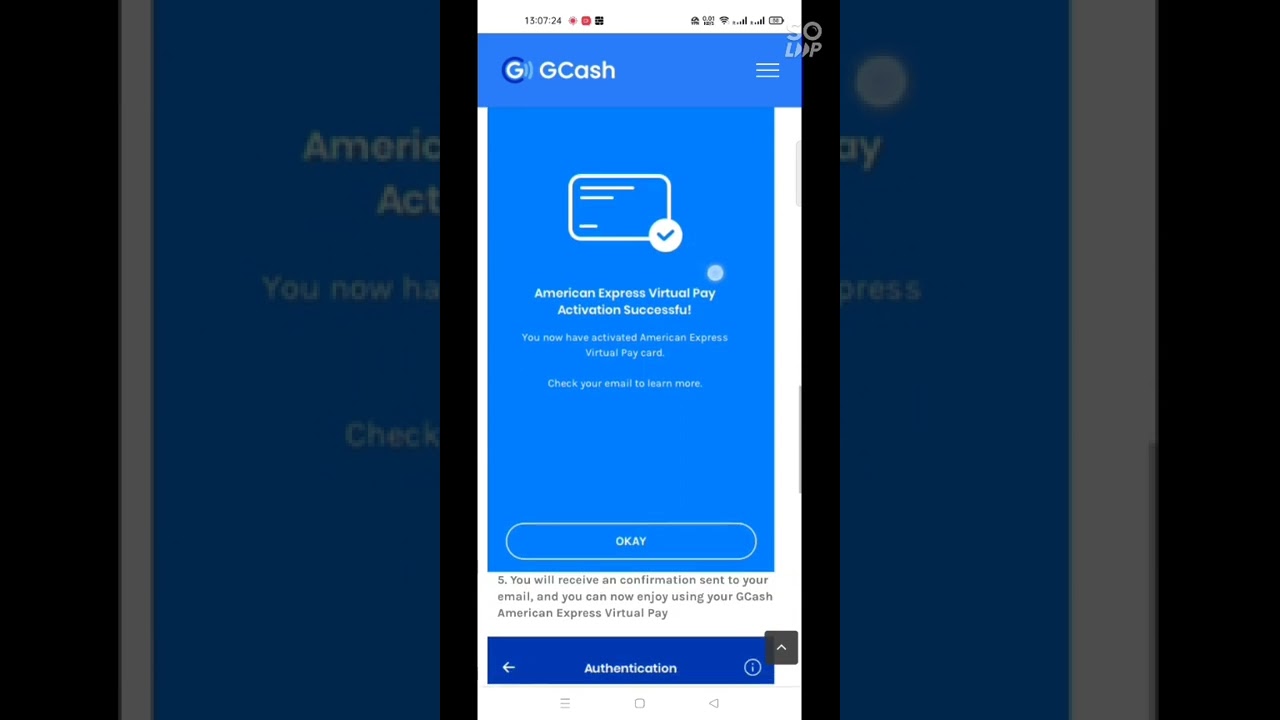**Descriptive Caption:**

The image is a detailed screenshot of a digital notification on a mobile phone within a computer screen, emphasized by the central portion being bright while the surrounding areas are grayed out. 

At the top of the screen, there is a standard status bar featuring the current date and a series of three icons next to it. Adjacent to these are icons indicating battery power and signal strength (depicted by two different sets of bars), along with additional icons in black.

Further down, the screen displays a blue area with the Google emblem, a blue circle with a white capital 'G' and light blue lines, followed by the text "GCASH" in white capital letters. Beside this text, there are three horizontal lines indicating a menu icon.

Below this section is a message indicating the successful activation of an American Express virtual pay card. The notification features a rectangular box with rounded corners, styled like a credit card. It has three lines of varying lengths simulating card information and a blue check mark within a circle at the bottom right of the card illustration.

The main message reads: "American Express Virtual Pay Activation Successful." Each word starts with a capital letter. Below this, another message states: "You now have activated your American Express virtual pay card." The instruction "Check your email to learn more" follows this in smaller text.

At the bottom of the notification is a bolded "OK" button in white capital letters against a blue rounded rectangle. Additionally, a small text in gray underneath states, "You will receive a confirmation sent to your email, and you can now enjoy using your GCASH American Express virtual pay card."

On the right-hand side of the screen, a vertical white bar runs from near the top to the bottom, featuring a black square with a white upward arrow, indicating further options or actions. To its left, there's a blue bar with a white leftward arrow and the word "Authentication" in white, accompanied by a small circular icon with a white ‘i’ on a blue background.

The bottom-most part of the background screen, which is white, shows three gray bars, a square, and what appears to be a small speaker or triangle pointing left. This suggests standard navigation or control icons.